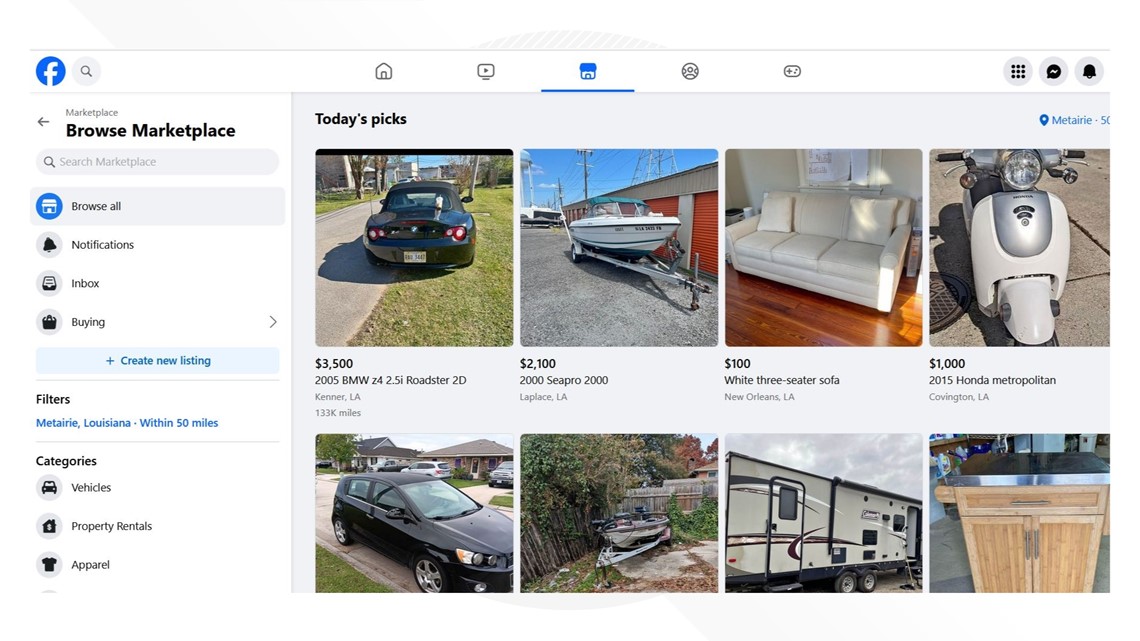This image captures a screenshot of the Facebook Marketplace interface. In the top left corner, we see the Facebook logo, a blue circle featuring a lowercase 'f'. Adjacent to it is a search icon represented by a magnifying glass. In the middle of the top bar are five prominent icons: a house, a movie reel, the highlighted marketplace icon resembling a storefront in blue, a sports ball, and an unfamiliar icon, followed by Messenger and notifications icons on the far right side.

Below the icons on the left, the menu for navigating the Marketplace is visible. The 'Browse Marketplace' option is bolded, with 'Browse All' currently selected. Other options such as Notifications, Inbox, Buying, and a 'Create New Listing' button in blue are listed below. Filter settings indicate a search within a 50-mile radius of a town in Louisiana, highlighted in blue. Categories chosen include Vehicles, Property Rentals, Apparel, and an area labeled 'Today's Picks' on the right side. 

The background of the interface is gray. Featured listings include, from left to right on the top row: a photograph of a BMW for sale, a boat for sale, a white leather sofa, and a Vespa scooter. The second row displays more items: another car, a boat, a camper, and what appears to be a vanity.